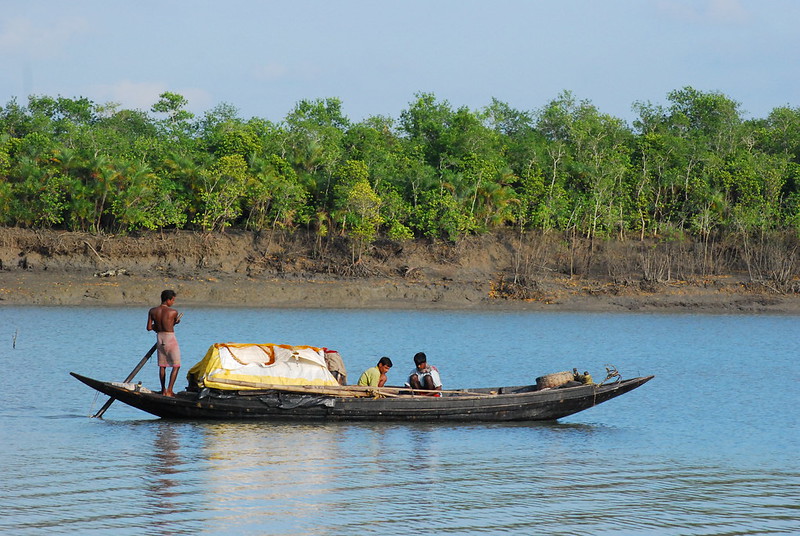The photograph captures a serene daytime scene by a river, showcasing a horizontal, rectangular image. At the top, a light grayish-blue sky stretches across, beneath which stands a horizontal row of medium-height green trees. The trees grow from a muddy, sandy shoreline with their roots visible in the wet dirt. The still waters of the river reflect the sky's blue hue, giving it a somewhat dark green appearance.

Dominating the center of the picture is a long, black wooden boat resembling a canoe or gondola, tapering to pointed ends. Standing at the back of the boat is a muscular, brown-skinned man wearing long, grayish board shorts. He is shirtless and holds a long brown pole in the water, suggesting he’s steering or pushing the boat forward. In front of him, a white and yellow tarp covers some goods stored in the boat.

Midway along the boat, two brown-skinned men are sitting, facing each other. Their positioning, along with the calmness of the water and the lush yet muddy riverside backdrop, adds to the tranquil yet industrious atmosphere of the scene.